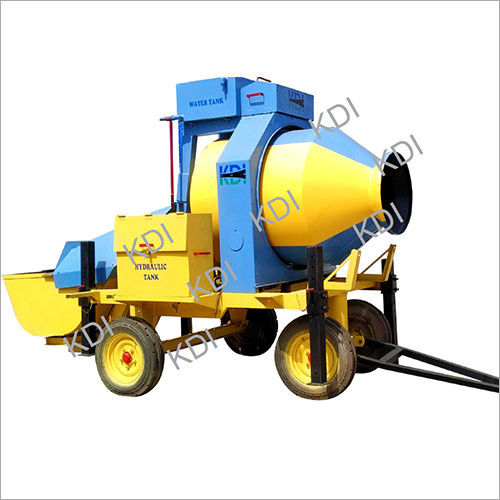The image depicts a bright yellow and blue mixing vehicle, likely used for cement mixing, set against a white background bordered by a thin black line. The vehicle features four yellow wheels with red hubs and a metal frame extending from the front wheels, suggesting it might be towed. At the front, a yellow bucket resembles the lifting mechanism of a bulldozer, while a box labeled "hydraulic tank" is affixed to the side, equipped with a handle crank. The mixer itself consists of a yellow and blue striped drum, surrounded by a blue metal frame labeled "water tank." Additionally, a black hole is visible near the right side of the mixer. The acronym "KDI" is prominently displayed in gray capital letters multiple times, both across the top and angled towards the right, as well as on the side behind the mixing drum.